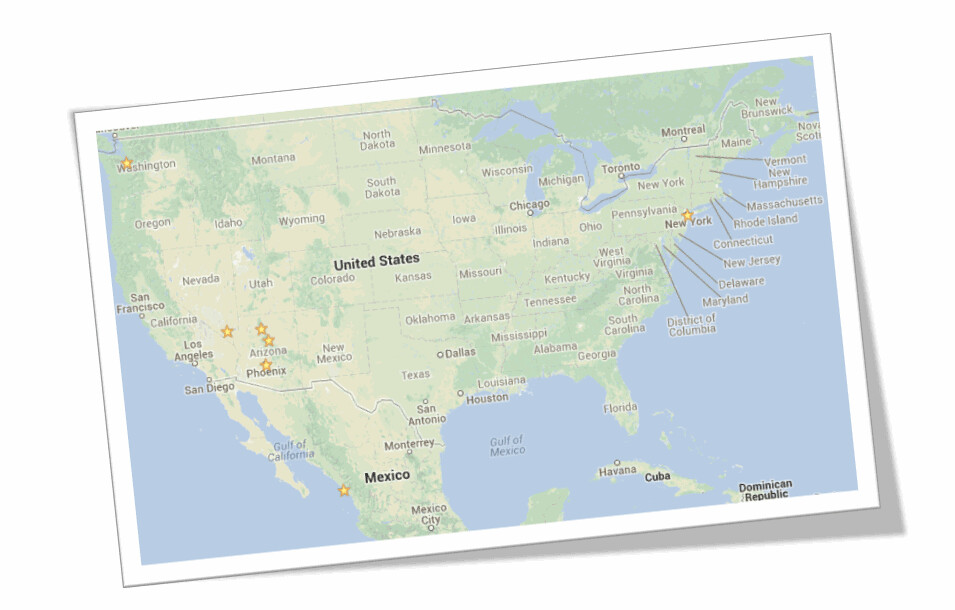This image depicts a detailed and slightly askew map of the continental United States, bordered by a white frame. The map includes major cities and states, with some cities in Canada and Mexico also named. The Gulf of Mexico is the only specifically named body of water, although both the Atlantic and Pacific Oceans are depicted in light blue. The map itself is a pale yellow with green interspersed, likely indicating landscape features, including mountain ranges shown in a darker brown. Additionally, parts of Mexico and Canada are visible, with the Great Lakes depicted in blue. Noteworthy locations like Cuba and the Dominican Republic can also be seen. Several stars mark notable locations, including one in Washington, one in Nevada, several in Arizona, possibly one in Utah, one in New York, and another in Mexico, which might be Acapulco.